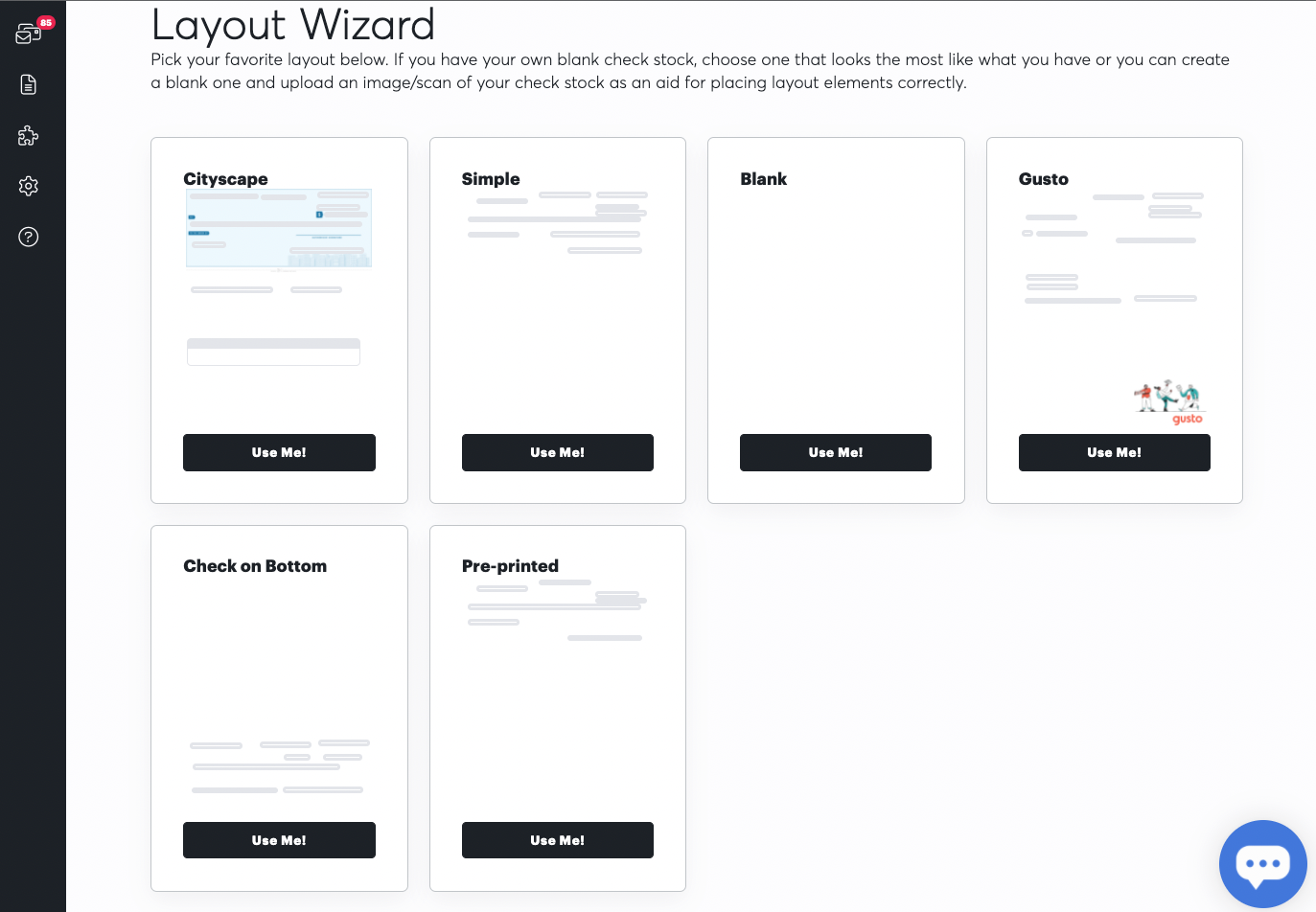The image displays a webpage for building a website, prominently labeled "Layout Wizard" at the top. Below this heading, there's a brief instruction or sentence. Underneath, there are several clickable options titled "Cityscape," "Simple," "Blank," "Gusto," and "Preprinted." Each of these options features a "Use Me" button, suggesting that these are different layout or theme choices for the webpage.

On the left side of the page, there is a blue border containing various icons arranged vertically. The top icon resembles an envelope, possibly indicating a Mail feature. Directly below is an icon depicting a document, suggesting a Page feature. The next icon, featuring a puzzle piece, appears to represent a Builder or customization tool. Following that is a gear icon, which likely leads to the Settings menu. The bottom icon is a circle with a question mark, indicating a Help or FAQ section.

The primary background of the page is white, while the borders and buttons are a dark navy blue, creating a clear and legible visual layout.